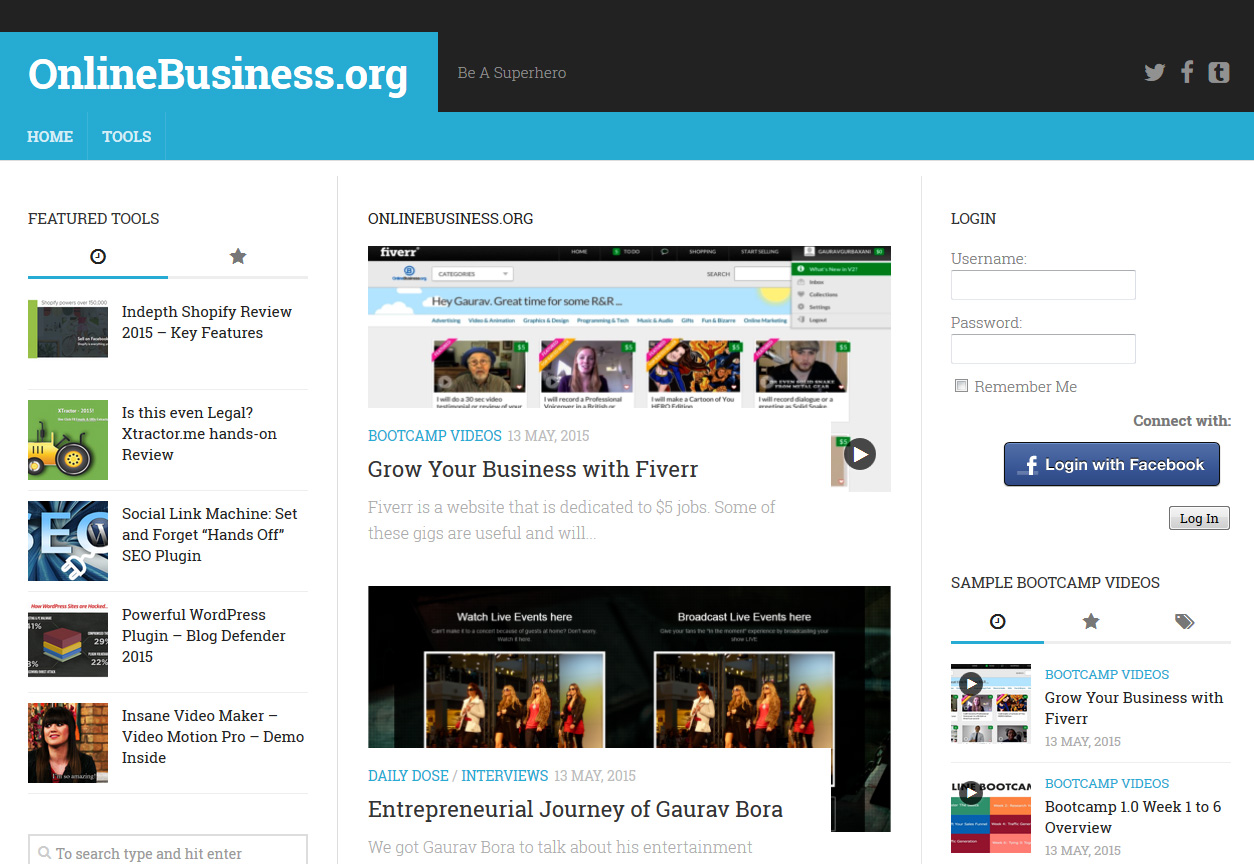This image is a detailed screenshot of a blog-like website, onlinebusiness.org. The website features a turquoise blue header with the website's name, "onlinebusiness.org," prominently displayed in white font in the upper left corner. Beneath it, a navigation menu includes options such as "Home" and "Tools." The right side of the header has a black strip with the phrase "Be a superhero" in grey font, accompanied by three grey social media icons: the Twitter bird, the Facebook "F," and a square with a black "T" representing Tumblr.

On the left sidebar, set against a white background, various categories are listed under the heading "Featured Tools." This section includes several review links such as "In-depth Shopify Review 2015" and "Is This Even Legal? Extractor.me Hands-On Review."

The central content area showcases the headline "onlinebusiness.org" in grey font, followed by a significant visual element—a screenshot from the Fiverr website. Beneath this screenshot, there is another headline in grey font that reads "Bootcamp Videos, 13 May 2015," indicating the content is from several years ago. An accompanying description in grey font reads, "Grow your business with Fiverr. Fiverr is a website dedicated to $5 jobs. Some of these gigs are useful and will..." before the text snippet cuts off.

On the upper right section of the website, there is a login area prompting users for their "Username" and "Password," with an alternative option to "Connect with" Facebook. Below this login section, there is a blue button labeled "Login with Facebook" in white font.

At the bottom right-hand corner under the bootcamp video headline, there are sample videos listed, each accompanied by small thumbnails, providing a visual preview of the content.

This detailed descriptive caption provides a comprehensive view of the various elements and layout of the onlinebusiness.org website screenshot.